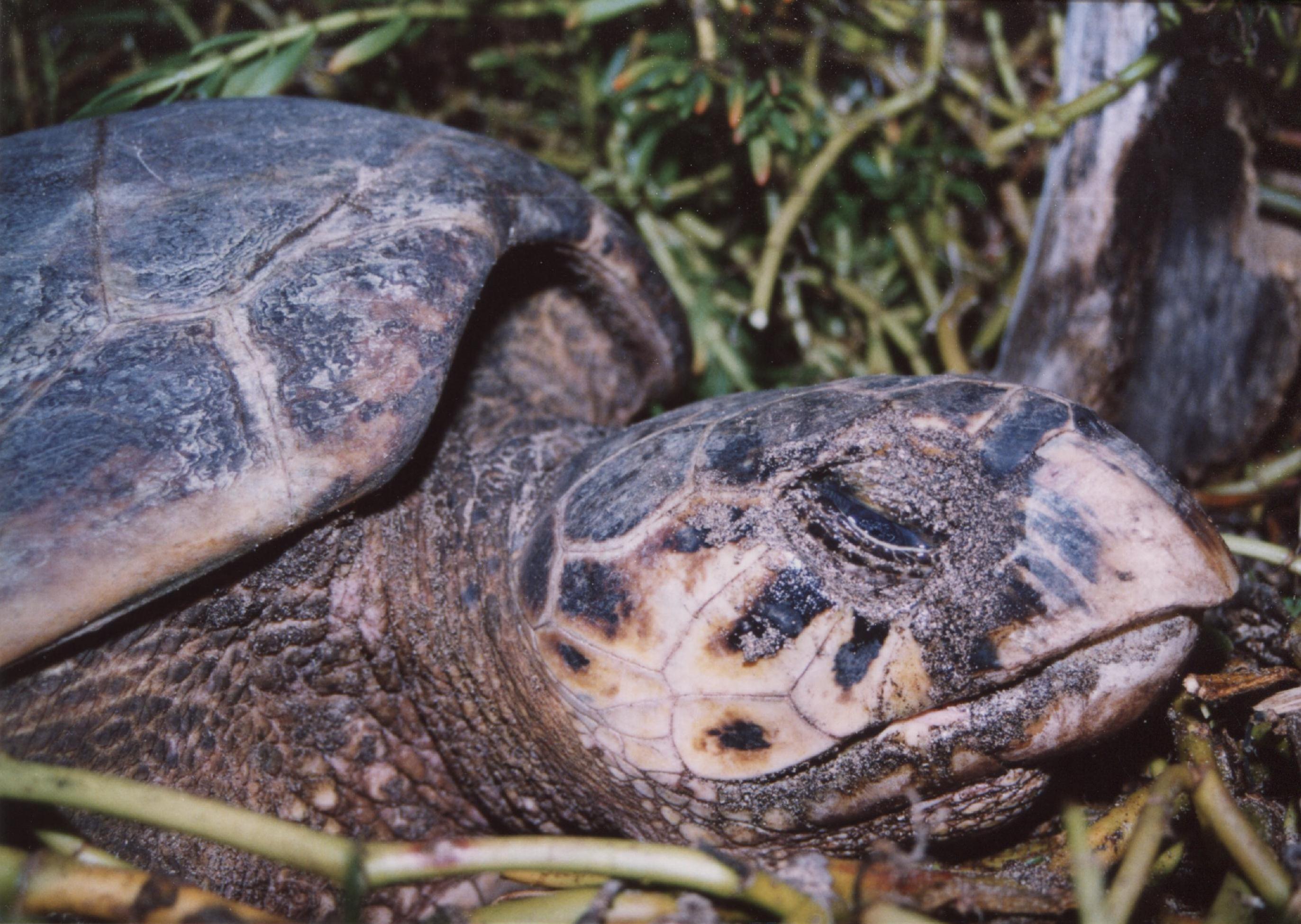The full-color square photograph, likely taken outdoors by a professional photographer, showcases an intricate nature scene. Dominating the image is a brown turtle, featured in profile with a hard, detailed shell and a slightly yellow beak. The turtle's head is extending out of the shell, revealing one half-closed black eye and a nose sticking out, with its closed mouth indicated by a visible line. The image captures not just the turtle, but also its surroundings: thick, wet, grass-like plants, a notable feature both at the top and the bottom of the frame. Some stems appear broken. In the upper right corner, there is a fragment of a log. Blaze grass and a leg of the turtle pointed out add to the rich texture and complexity of the scene.